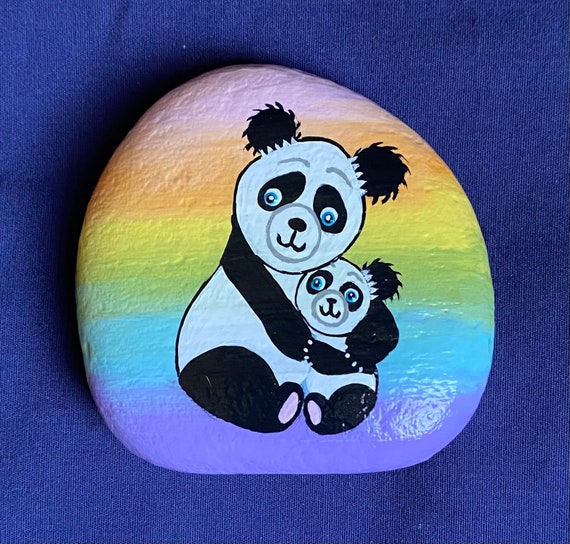In the image, a multicolored, slightly curved stone with a flat base and a sharp top edge lies on a blue, jean-like fabric surface. The stone is adorned with a detailed painting of a mother panda holding her baby panda on the left and right, respectively. The pandas are characterized by their black ears, arms, and necks, with the mother panda embracing the baby closely. Both pandas feature blue eyes, white paws, and the baby appears to be smiling while the mother exudes a protective demeanor. The stone's background transitions through a vibrant spectrum of colors from bottom to top: purple, blue, green, yellow, orange, and pink, contributing to the rock's shiny and bright appearance.